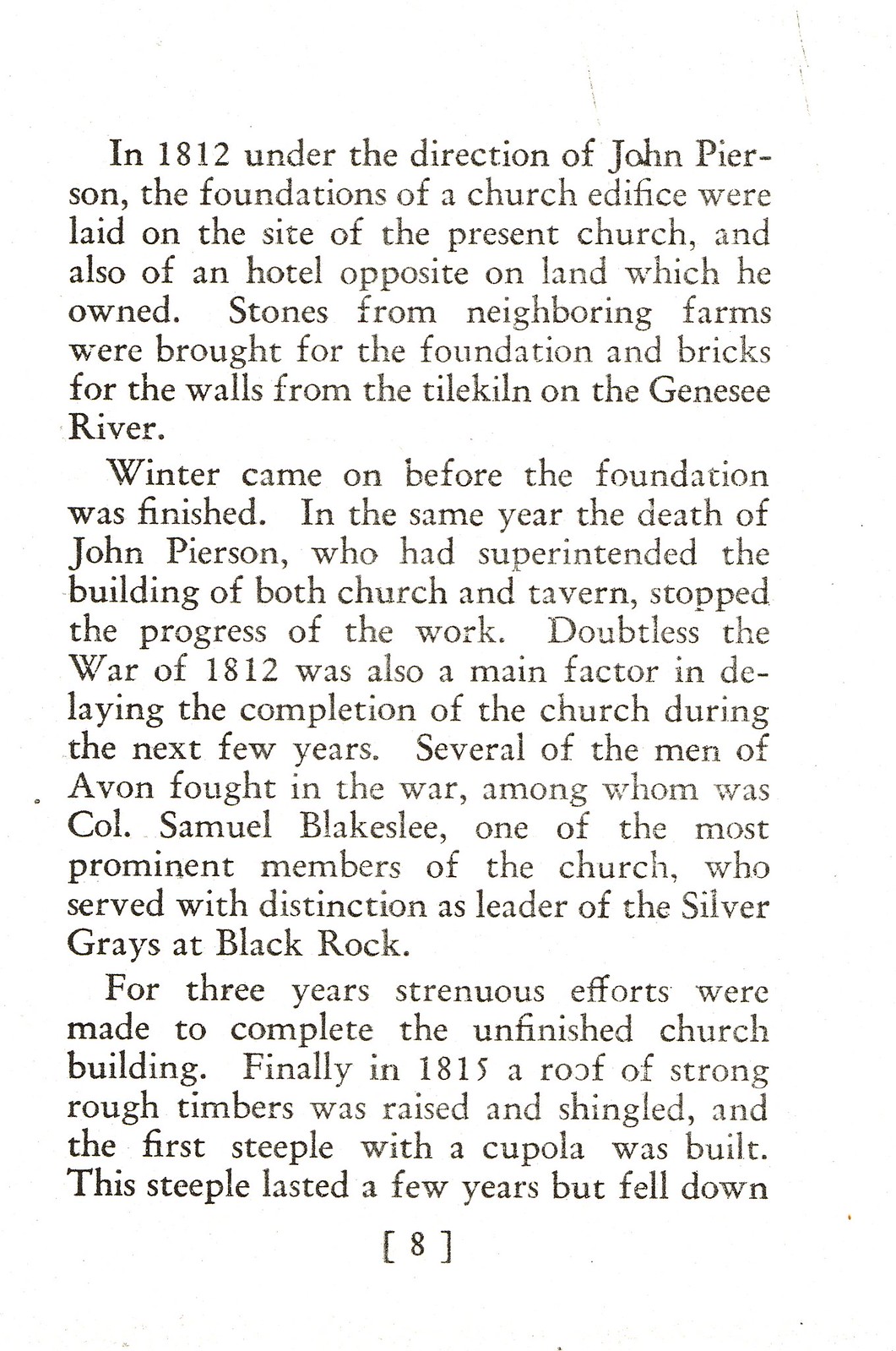This image is a black and white digital screenshot showcasing an excerpt from a book, specifically page 8 as indicated by the number at the bottom. The background is white with black text, which spans three paragraphs. The passage begins with "In 1812, under the direction of John Pearson," detailing the establishment of a church edifice and a hotel on land owned by Pearson. The text describes the construction process, noting that stones were sourced from neighboring farms for the foundation and bricks from the Genesee River area for the walls. Unfortunately, winter halted progress, and the death of John Pearson that same year further delayed the project. Additionally, the War of 1812 significantly impeded the church’s completion, as many local men, including Colonel Samuel Blakeslee, a prominent church member, were enlisted in the war. The excerpt continues but the provided text ends, leaving the story of the church unfinished.